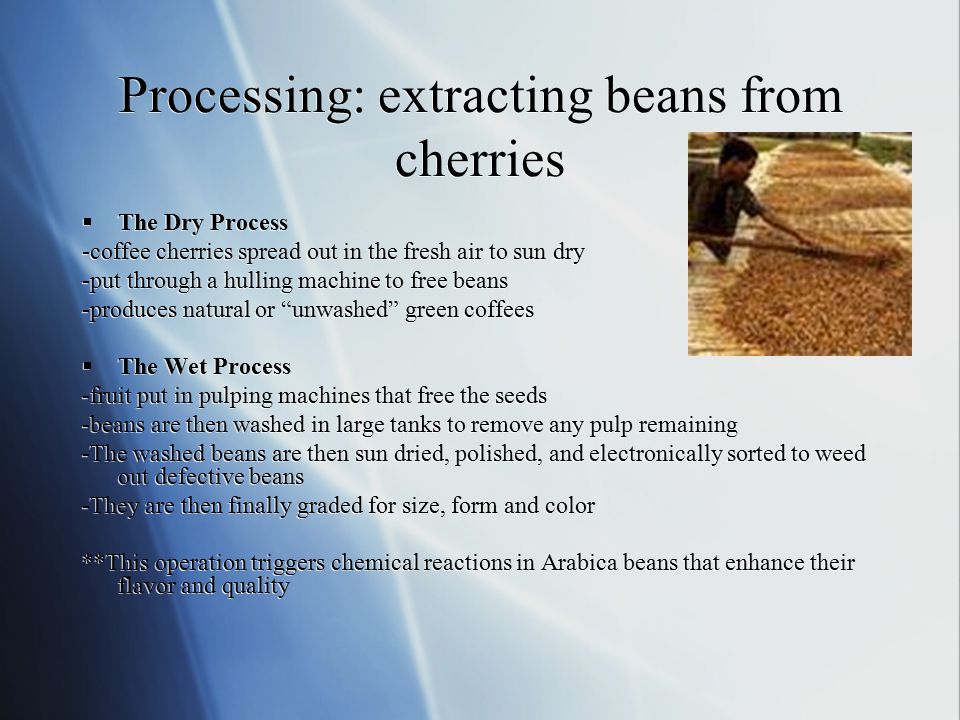The image is a slide from a PowerPoint presentation titled "Processing: Extracting Beans from Cherries." It details the dry and wet processes of coffee bean extraction. In the dry process, coffee cherries are spread out in the fresh air to sun-dry before being put through a hulling machine to free the beans, resulting in natural or unwashed green coffees. The wet process involves pulping machines that free the seeds, followed by washing the beans in large tanks to remove any remaining pulp. The washed beans are then sun-dried, polished, and electronically sorted to remove defective beans, and finally graded for size, form, and color. This operation triggers chemical reactions in Arabica beans that enhance their flavor and quality.

The slide features a smaller image in the top right corner showing a man holding a stick, working with coffee beans laid on the ground. The coffee beans are light brown in color. The background of the slide transitions horizontally from dark blue to pale blue, with black text on top and bullet points detailing the processes. The overall visual style suggests an informational piece, likely used for educational or training purposes.